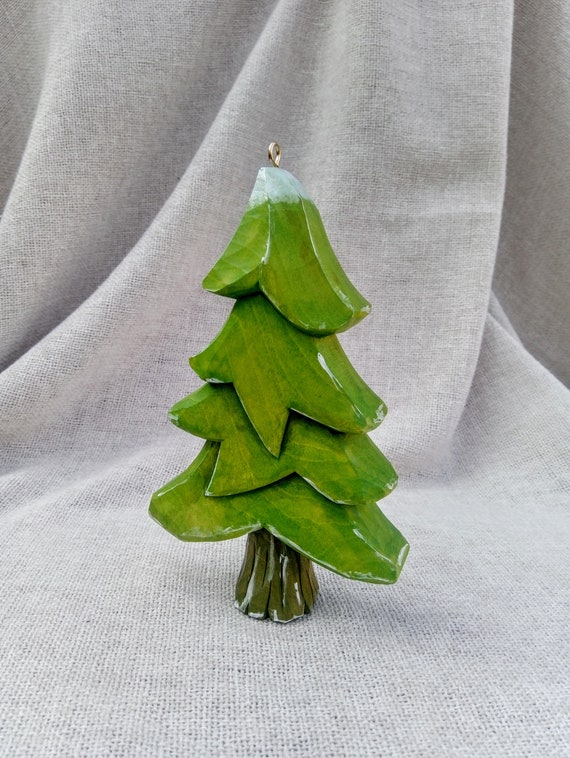The image depicts a meticulously crafted evergreen tree ornament, designed to be hung using a small gold loop at its top. The tree is likely made of wood or possibly ceramic and consists of four solid blocks stacked to resemble sloping branches. These branches are painted a rich green, giving the appearance of natural foliage. The top of the tree is lightly frosted with white paint, simulating snow that has freshly fallen, with a subtle dusting of white also visible near the trunk, which is primarily brown. This ornament rests on a gray fabric that lies flat at the bottom of the image and drapes upward toward the top, providing a neutral backdrop that emphasizes the intricacy of the tree design. The background further enhances the focus on the ornament, which captures the essence of a snow-kissed Christmas tree awaiting to be part of festive decorations.